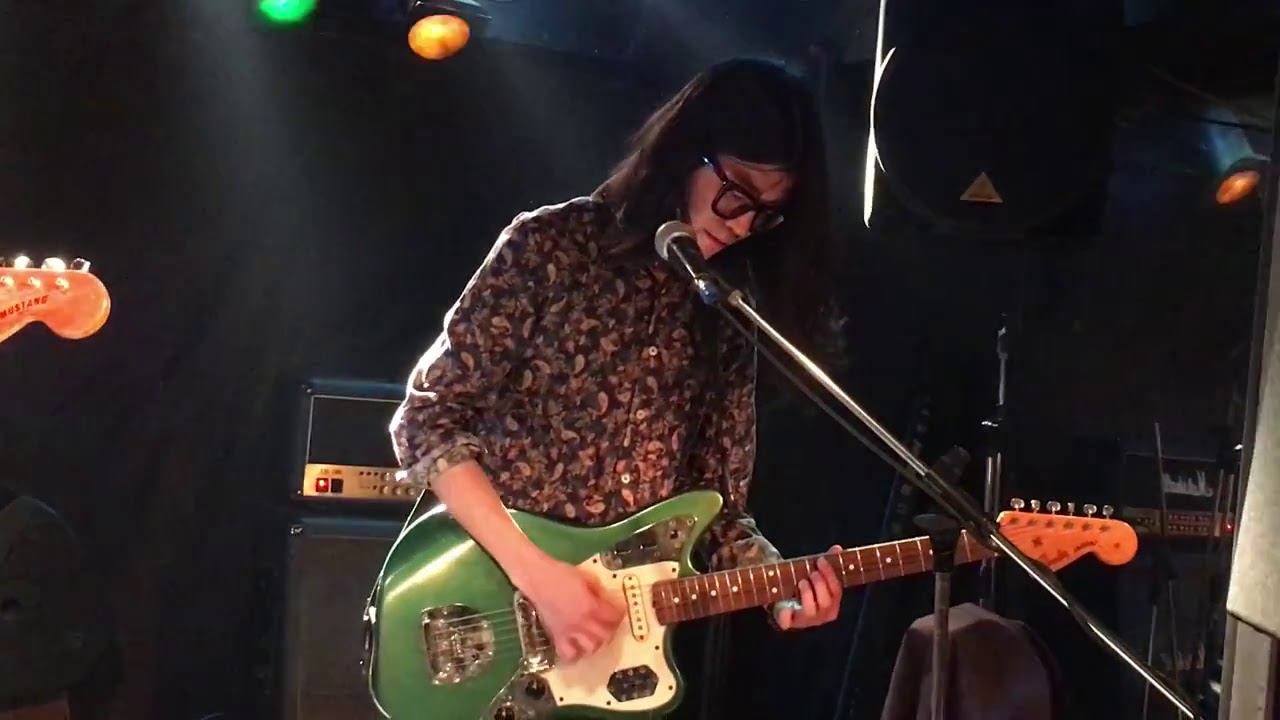In this image, we see an Asian guitarist with long, dark hair, wearing thick glasses and a floral or paisley-patterned, long-sleeve button-down shirt. He stands in front of a silver and black microphone, performing on stage. He is playing a green guitar with metal components, including metal strings, knobs, and an orange handlebar at the end. His left hand holds the guitar’s neck, while his right hand strums the strings. The background is mostly black, and the stage is illuminated by spotlights emitting green, yellow, and orange hues, creating a smoky ambiance. Behind him, several amplifiers, including blue and black ones with red lights, and Marshall brand amps are visible. There is also the neck of another guitar, labeled "Mustang," protruding from the right side of the frame, indicating the presence of another musician nearby. The guitarist appears deeply focused on his music, looking intently at his finger placement on the guitar.